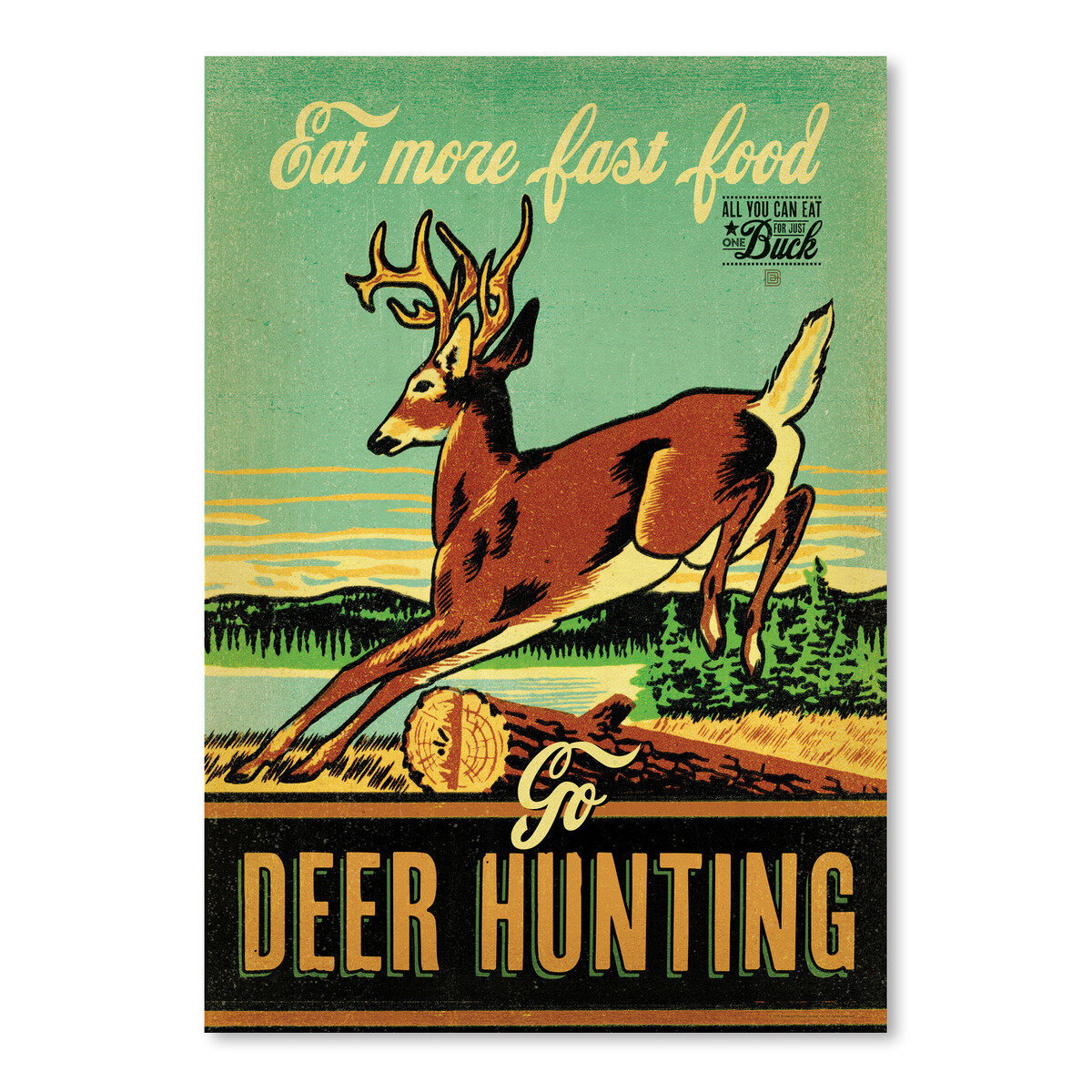This image appears to be a vintage-styled advertisement for deer hunting, reminiscent of a retro magazine cover or poster. At the top, in yellow cursive text, it boldly declares, "Eat More Fast Food." Beneath this, in the upper right corner, is the additional text, "All you can eat for just one buck," with the word "four" in a small font positioned between a star symbol and the number one. The central focus of the image is a striking illustration of a brown buck mid-leap over a cut log, its back feet suspended in the air while its front feet stretch forward, just about to land. The log it clears has clean, straight-cut sections and a single truncated branch. The background showcases a picturesque landscape with a dense row of pine trees close on the right, extending into more distant hills and a serene lake. At the bottom, in orange block letters accented with a green shadow, it commands, "Go DEER HUNTING." The timeless retro aesthetic of this ad, likely from the 1940s, merges nostalgia with the rugged allure of the great outdoors.